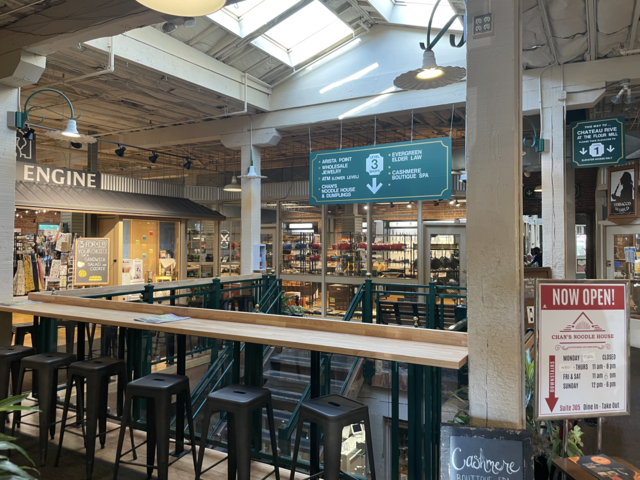The image shows the interior of a multi-level mall with a focus on its upper floor, presumably the third floor based on the sign that reads "Third Floor" prominently displayed at the entrance of a staircase. The staircase, centrally located in the image, ascends to the vantage point from which the photo is taken. Arrayed in a square layout, various stores and eateries border this upper floor. To the left, there is a clothing store named "Engine," identified by its white text sign and a chalkboard at its entrance with some written details. Near this store, a chalkboard announces the opening of "Chan's Noodle House," situated close to a bar area equipped with black stools and a wooden countertop. The ceiling above is pitched and features windows that allow natural sunlight to illuminate the space, supported by structural posts that appear to be either brown-painted steel or wood. The bustling atmosphere is further emphasized by the abundance of seating areas with tables and chairs, indicating a possible food court area.